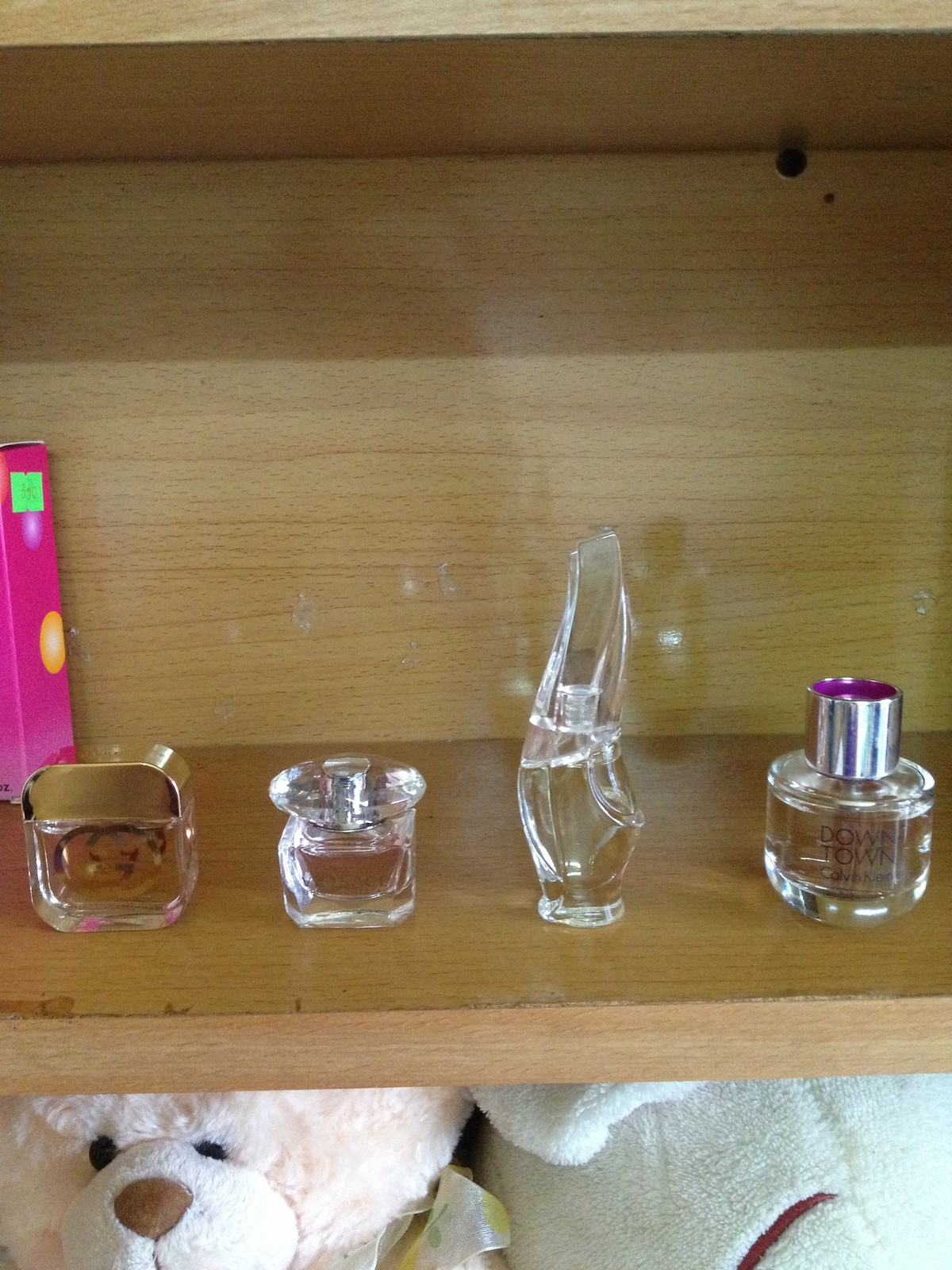The image features a wooden shelf that appears to be protruding from the wall. This shelf is the focal point and displays four distinct perfume bottles, each uniquely shaped. The bottles are relatively similar in size, but vary in design: the first on the left is clear with a brass lid, the second is a clear glass bottle with a round top, the third is slightly taller with a curved silhouette, and the fourth resembles a nail polish bottle with a silver top and a hint of purple color on its lid. Additionally, there is a taller, pink-colored box with a little green sticker and a yellow circle on it situated to the left of the perfume bottles. Notably, beneath the shelf, the faces of two stuffed animals are visible: a pink teddy bear with a brown nose and black eyes, and another white stuffed animal that is partially obscured.